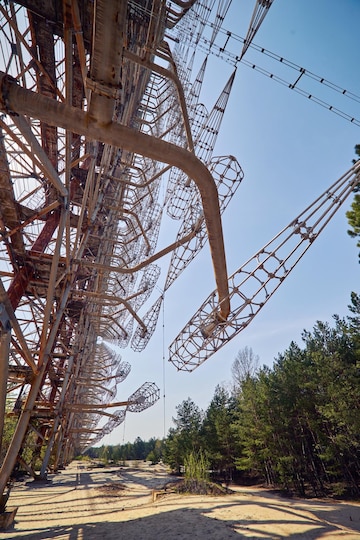The image depicts an outdoor scene during the daytime, with a clear blue sky. On the right-hand side, there are rows of green evergreen trees, possibly pine, extending into the distance along a dirt-covered or sandy path. Prominently on the left side of the image is a large, steel structure made of rusty gray metal. The structure has scaffolding-like steel beams that extend outward, with various metal pipes and wire-mesh cages attached, resembling thin, conical shapes. These elements are suspended in the air, and the structure looks complex and possibly engineered, though its purpose is unclear. There are no people visible in the photograph. The overall scene combines elements of nature and industrial design.